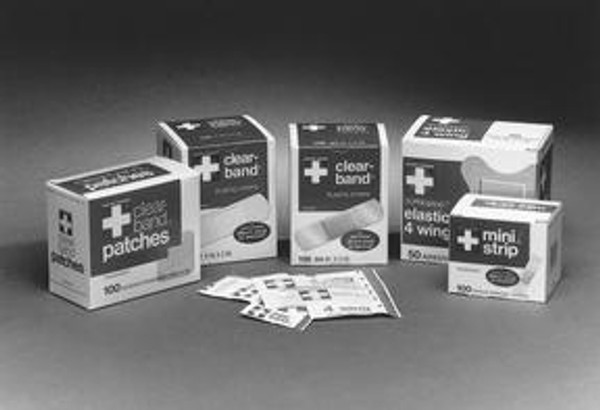A black-and-white photograph showcases a collection of vintage band-aid and first aid item packages, arranged on a gradient background that transitions from black at the top to lighter shades at the bottom. Five distinct boxes, displaying a slight curved alignment, each prominently feature a white cross logo. The individual boxes are labeled: the first one on the far left says "Patches," followed by "Bands," "Clear Band," "Elastic Four Wings," and finally "Mini Strip" on the far right. Each box differs slightly in size but collectively encapsulates various types of bandages. In front of these boxes are several loose bandage packets, still enclosed in their paper coverings, providing a glimpse of the products inside without revealing the actual bandages. The overall scene gives a nostalgic look at first aid packaging and branding.